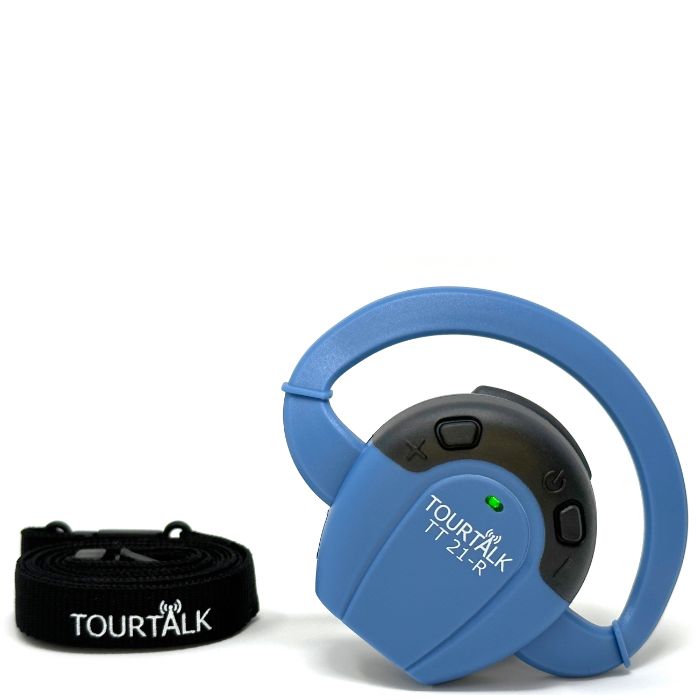In the image, we see two distinct objects arranged side by side. 

On the left is a sleek, all-black headband-like device, likely a 3D or VR headset. The headband features small rings on its back end, possibly designed for hanging or adjusting. Prominently displayed on the front circular band is the brand name "TOR TOC" in bold, white uppercase letters. Notably, the letter "A" in "TOR TOC" is stylized with a small extension on its tip, flanked by two wave-like lines, resembling a signal tower symbol.

On the right side of the image is a wheel-shaped object with a handle oriented on the upper right half, slanting slightly upward. The inner portion of the wheel is black, contrasting with the predominantly blue body of the wheel. At the center of the wheel, there's a small green rectangular dot. Below this, the same brand "TOR TOC" is printed, followed by the model number "TT21-R."